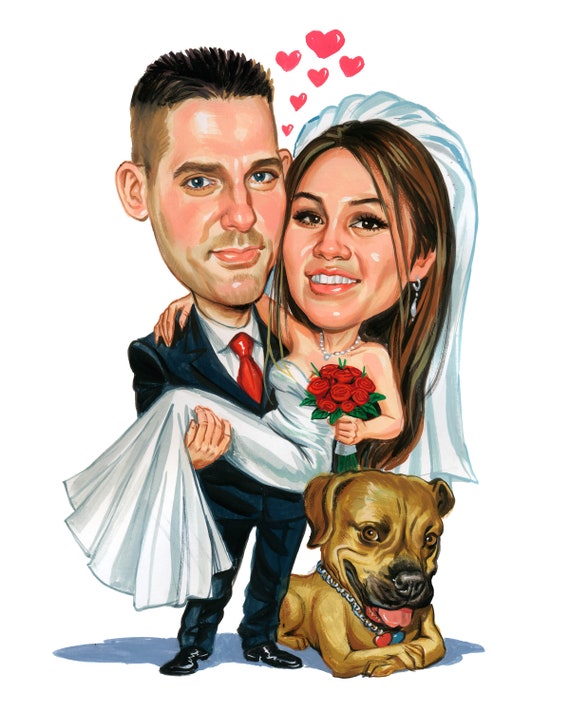The image is a cartoon-style drawing of a bride and groom on their wedding day, depicted with exaggeratedly large heads and small bodies. The groom, who sports a very short haircut, is wearing a navy blue suit paired with a red tie and a white shirt. He is lovingly carrying the bride in his arms, creating a romantic scene. The bride, draped elegantly in a long, sleeveless wedding dress, has her right arm affectionately wrapped around the groom's neck. She holds a bouquet of red roses and is adorned with a pearl necklace, pearl teardrop earrings, and a wedding veil that flows behind her head. Both the bride and groom have light brown hair and are depicted as Caucasian. Between their heads, a series of small red heart symbols float upward, accentuating the love between them. Beneath the couple lies a golden brown dog, also rendered in a cartoon style with a big head, sporting a chain-link collar with red and blue heart-shaped tags and its tongue playfully hanging out.